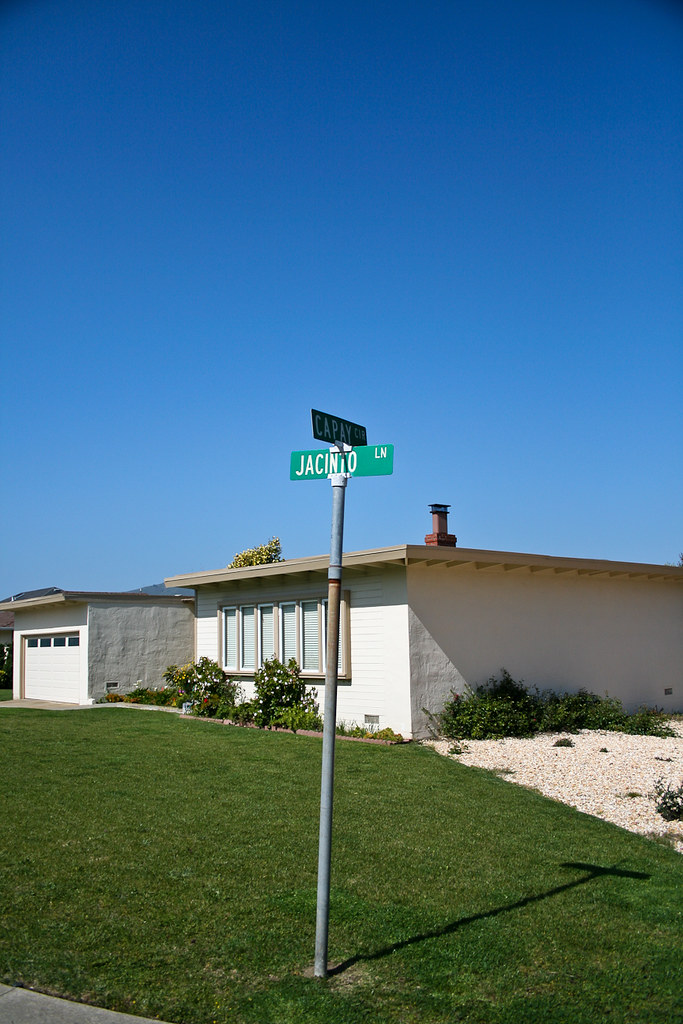This photograph captures a charming one-story house situated on a corner lot under a clear, blue sky. The house, constructed from a pale beige stuccoed brick, features a flat roof with an extended edge and visible beams. A distinct red metal chimney topped with a black cap punctuates the roofline. A well-maintained green lawn sprawls in front of the house, accompanied by a landscaped flowerbed and various plants and bushes that hug both the front and side of the structure. The house includes a two-car garage with windows, separated from the main building by a walkway.

Flanking the intersection, a metal street sign pole with a dull finish displays the names "Jacinto Lane" and "Capay Circle." Below the sign, lush green grass contrasts with the light concrete curb at the bottom left corner of the image. A gravel bed with brown rocks is visible at the corner of the house, highlighting the meticulous landscaping. A small tree peeks over the roof, adding to the picturesque suburban setting.